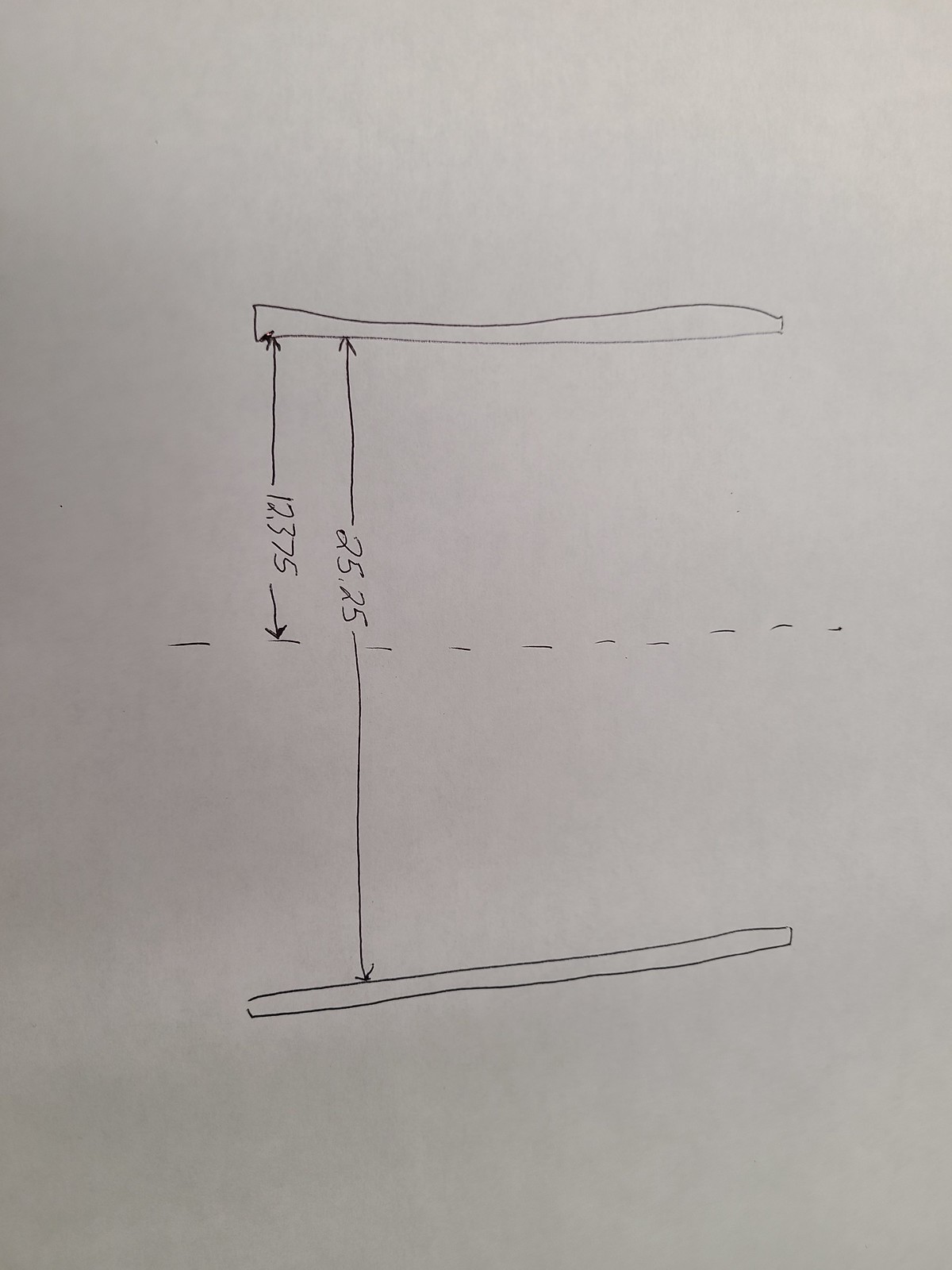This image features a rough sketch representing measurements between two thin, non-parallel rectangles, possibly signifying walls or boards. The drawing includes labeled distances with explanatory arrows. A dashed line divides the rectangles, illustrating a midpoint. The distance between the top rectangle and this dashed line is marked as 12.375 units, denoted by a line drawn from the number to the top rectangle and the dashed line. Similarly, the measurement between the top and bottom rectangles is indicated as 25.25 units, with a line extending from the number to both rectangles, marked by arrows at each end to clarify the distance.